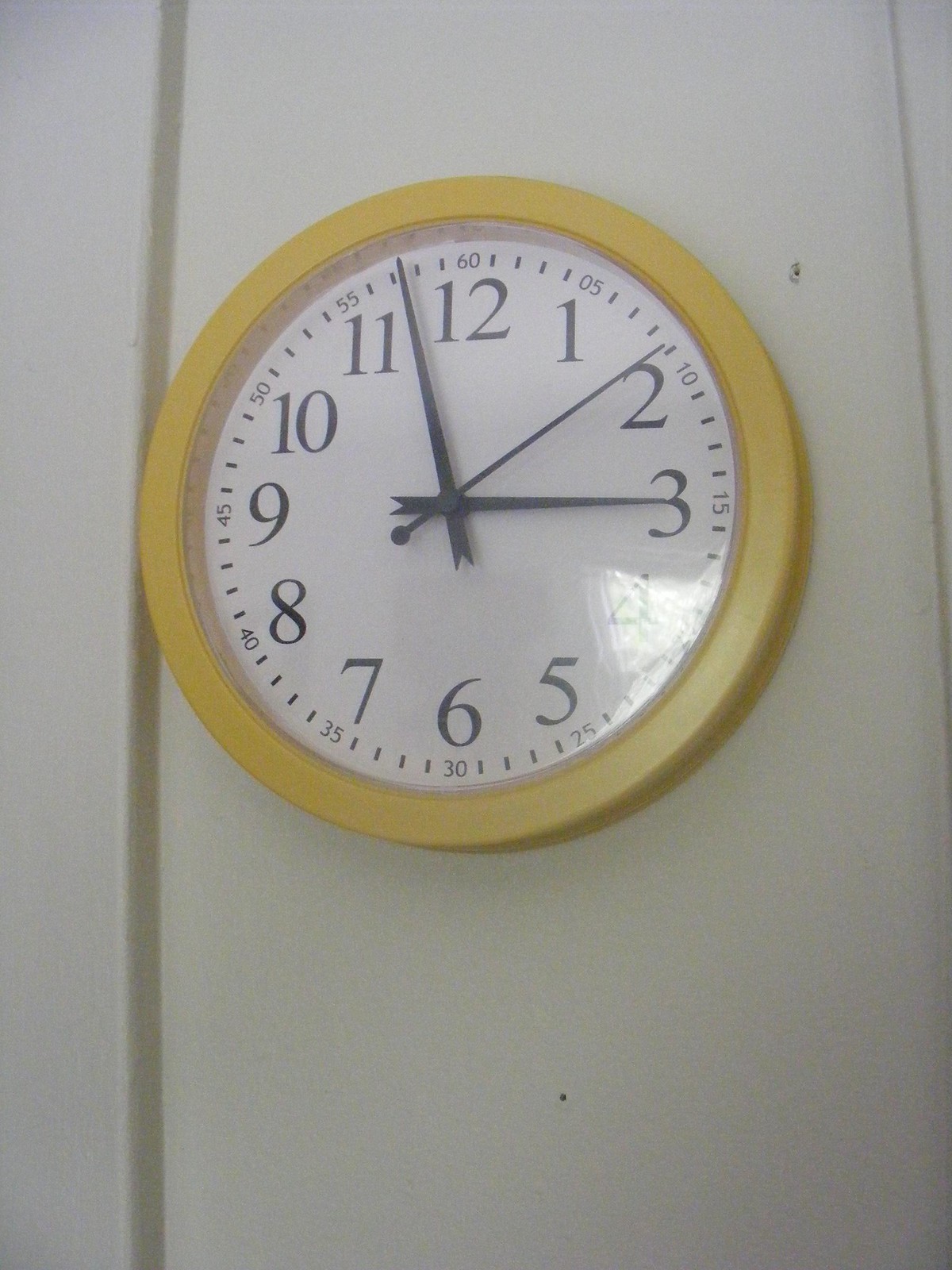The image features a possible exterior wall composed of white painted boards. Mounted on this wall is a prominently displayed circular clock. The clock's rim is painted in a bright yellow hue, contrasting sharply with its white face. The clock hands are simple yet distinct, with the hour and minute hands shaped as elongated black triangles and the second hand designed as a straight black indicator, adorned with a small ball on the opposite end. The clock is numbered from 1 to 12, with minute markers indicated by ticks and numbers every five minutes (e.g., 05, 10, 15, 20, 25). The current time displayed on the clock is precisely 2:58 and 8 seconds.